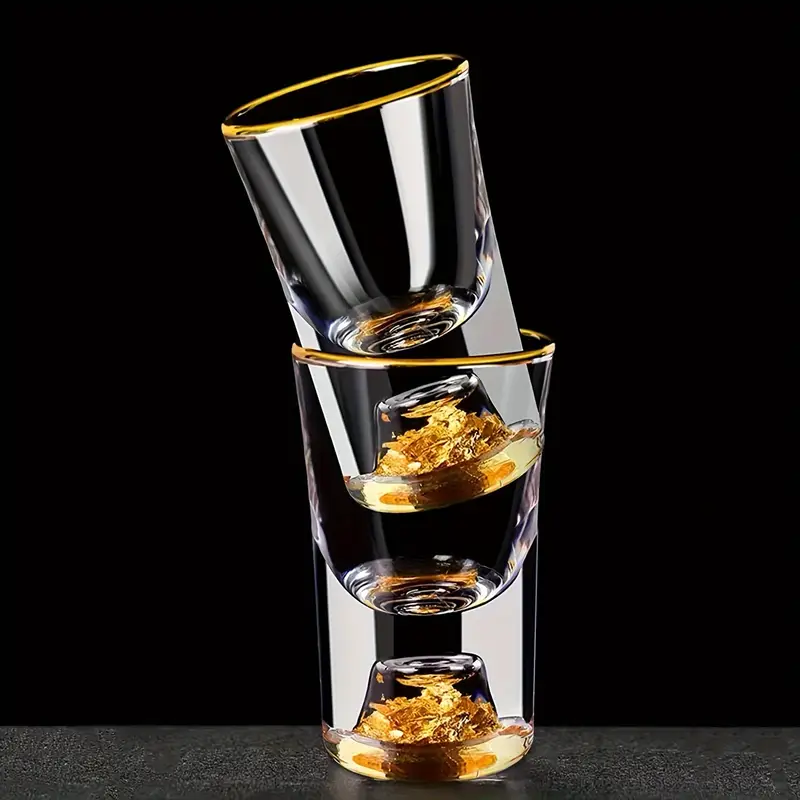The photograph features two clear shot glasses, one resting inside the other at a slight angle towards the top left corner. The glasses are positioned on a dark grey surface against a solid black background. Both shot glasses have distinctive gold rims and contain golden flecks in a small chamber at their bottoms. The outer glass stands straight, while the inner glass is slightly tilted, creating an overlapping effect that showcases the intricate details of their design. The glass surfaces are shiny, suggesting they are either new or meticulously clean, further accentuating the brilliance of the gold accents.